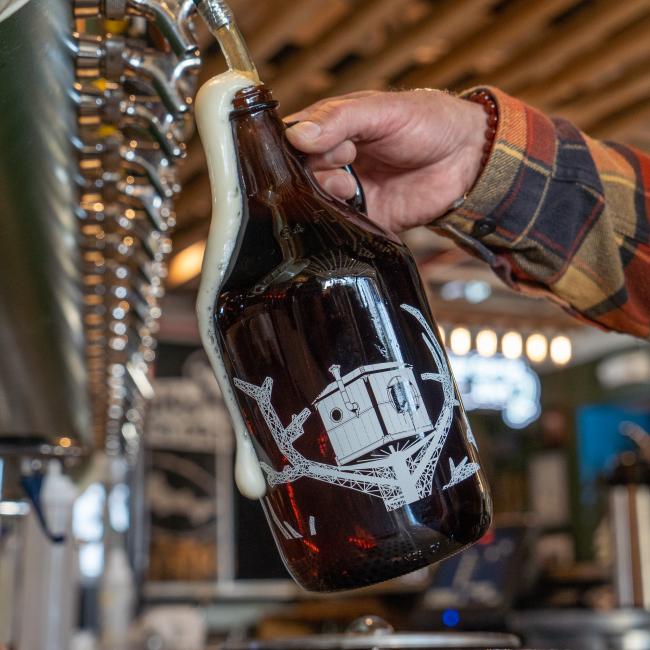The photograph captures a detailed scene of a man filling a brown beer growler from a series of beer taps in what appears to be a restaurant or brewery. The man's rough, hairy hand, adorned with a bracelet of brown spheres, firmly grips the jug's handle while white foam spills over the front of the growler. The growler features an intricate white design resembling a treehouse with a chimney and a round window. The man is dressed in a plaid jacket with hues of orange, brown, green, blue, and yellow. The dispenser system consists of multiple spigots extending into the background, gradually blurring with distance. Behind the row of taps, the setting remains slightly out of focus, revealing hints of neon signs, ceiling lights, and other restaurant patrons.